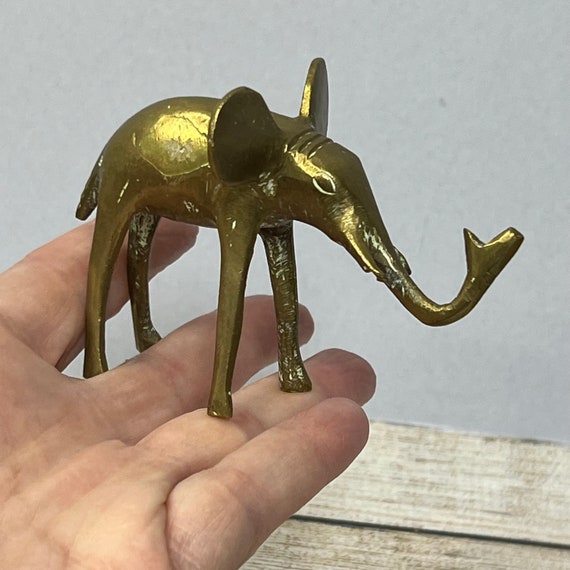In this photo, a left hand is holding a golden, slender elephant figurine with remarkably long, giraffe-like legs. The sculpture, which appears solid and heavy despite its delicate form, features disproportionately large ears reminiscent of a mouse, a long curving trunk, and detailed engravings including eyes and tusks. The background consists of a grey wall and a light-colored wooden surface, creating a contrast that highlights the figurine's dark gold color.